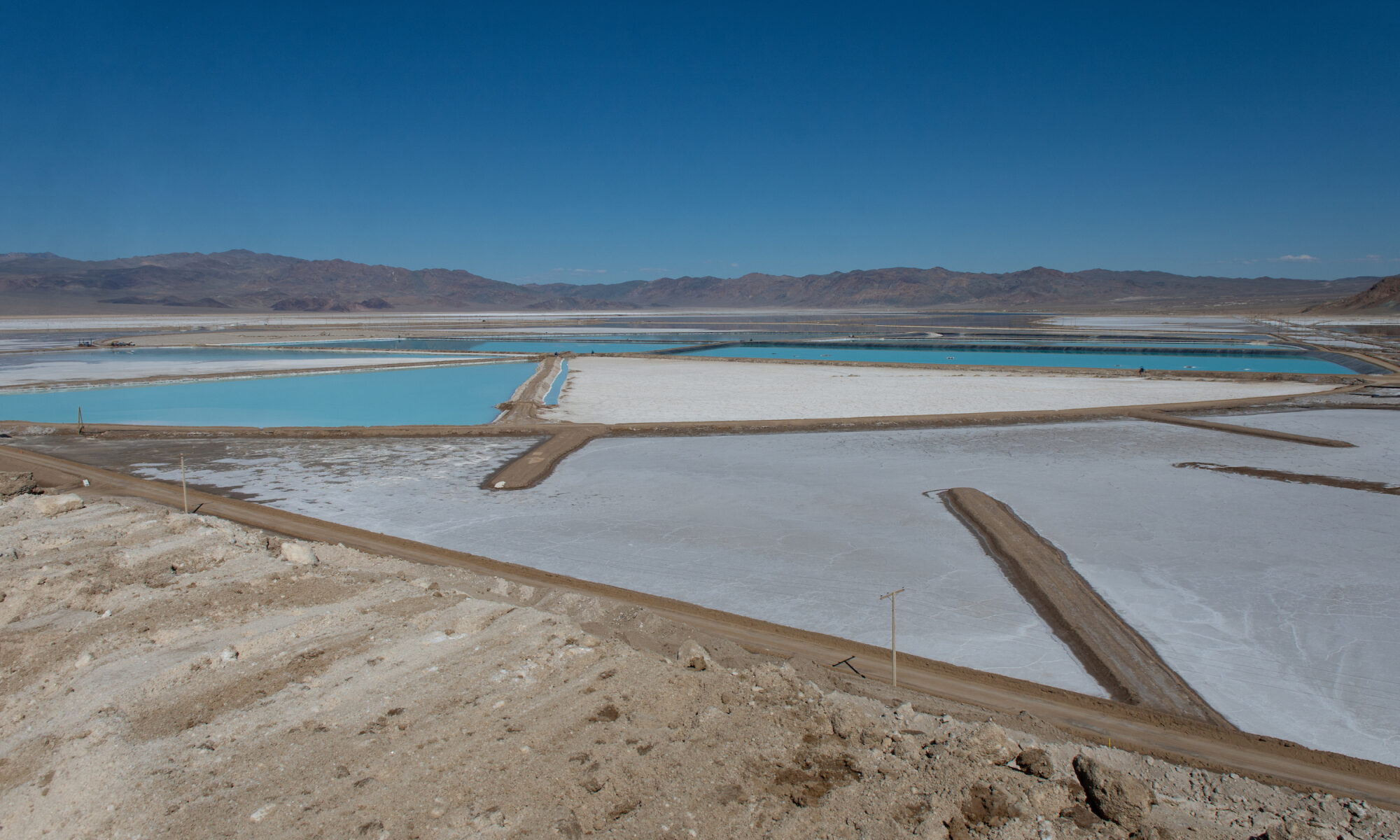The image depicts an outdoor landscape with a clear and vibrant blue sky that darkens as it extends upwards, occupying the top third of the frame. Below the sky, a distant mountain range stretches thinly across the horizon with subtle reddish-brown hues. Dominating the lower portion of the image is a body of water visible in the distance, surrounded by varying terrains. In the lower left corner, a triangular area of dirt and rocks blends into the scene, intersected by a brown dirt road. This road, lined intermittently with telephone poles, meanders through the landscape, cutting through an area filled with what appears to be gray material, likely a retention ditch or some kind of containment area. Adjacent to this gray section, another distinct triangular section appears to be filled with a white substance, resembling concrete. Flanking this structure, there are areas filled with light blue material, presumably water, echoing the blue tones of the sky above. The intricate network of roads and the arrangement of various containment sections suggest a well-structured landscape captured from a high viewpoint, possibly a drone, offering a comprehensive overview of this striking outdoor scene.